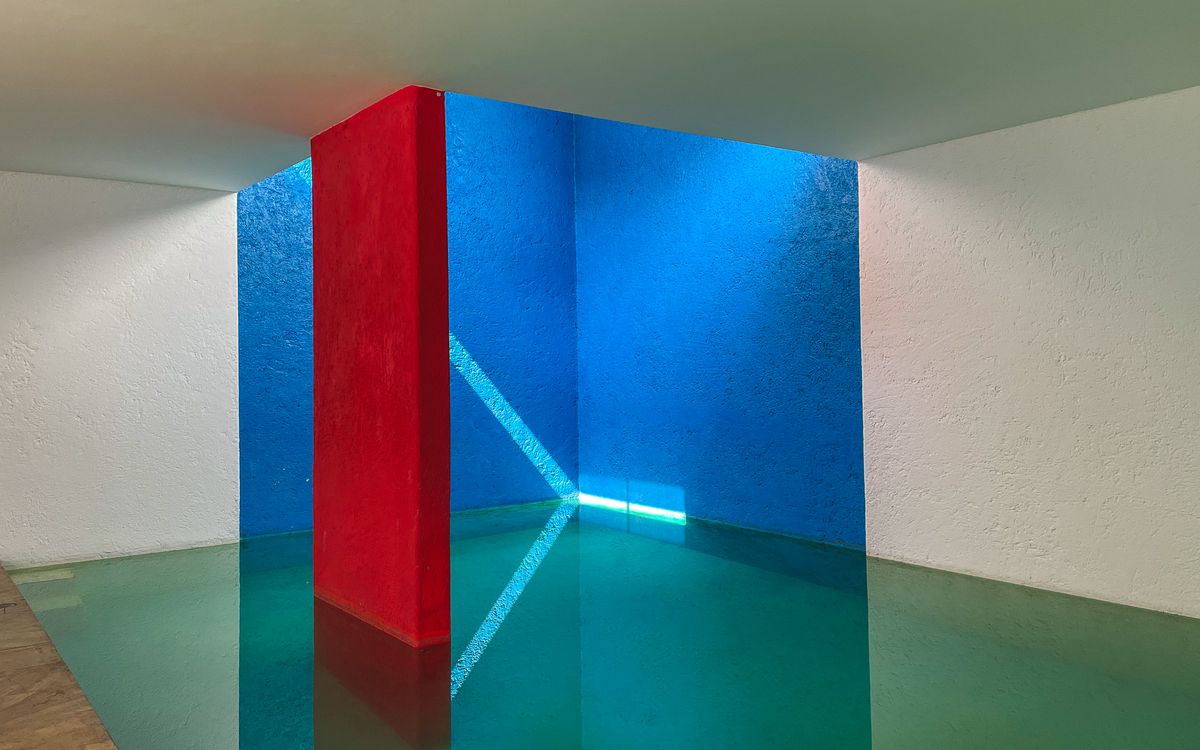This image captures a corner of a room where an intriguing blend of colors and materials dramatically contrasts with the white walls. The corner itself is vividly painted in bright blue on both the left and right sides, while a striking raspberry-red post extends from the floor to the ceiling on the left. A crisp white line is drawn on the left blue wall, spanning diagonally to the bottom right of the adjacent blue wall, and further extends into the glossy, green sea glass-like flooring, which appears smooth and reflective, adding depth and dimension to the space. Light streaming into the corner casts a soft, turquoise hue, while the rest of the room, including the ceiling, remains shadowy. This artistic composition creates a visually stunning and dynamic contrast, making the corner particularly eye-catching amidst the predominantly white surroundings.